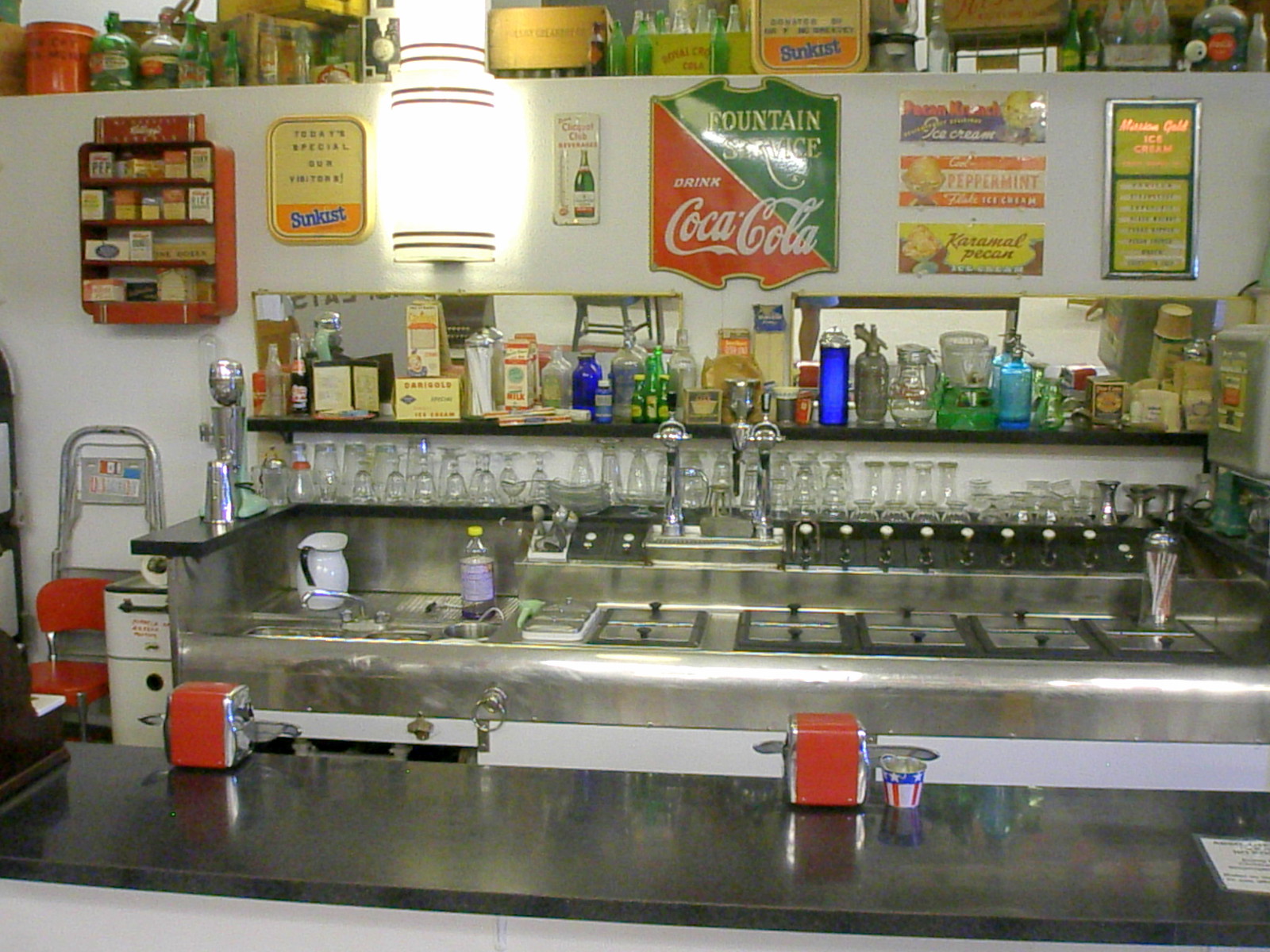The image depicts a cozy, vintage diner or cafe interior. The central focus is on a gleaming, dark marble countertop adorned with red napkin dispensers and a small cup featuring stars and stripes. Embedded in the stainless steel counter are several built-in compartments with lids, likely for food or ice cream storage. Along the back wall, there is a shelf lined with neatly arranged wine and drink glasses. Above the glasses, the shelf holds various large bottles and items. The white wall behind this setup is decorated with colorful advertisements, including a prominent green and red "Fountain Service Drink Coca-Cola" sign and a "Sun-Kist" poster. A bright white light illuminates the area, enhancing the nostalgic ambiance. To the left, a red seat adds a pop of color to the scene. The overall setting suggests an inviting ice cream or soda pop bar with a retro charm.